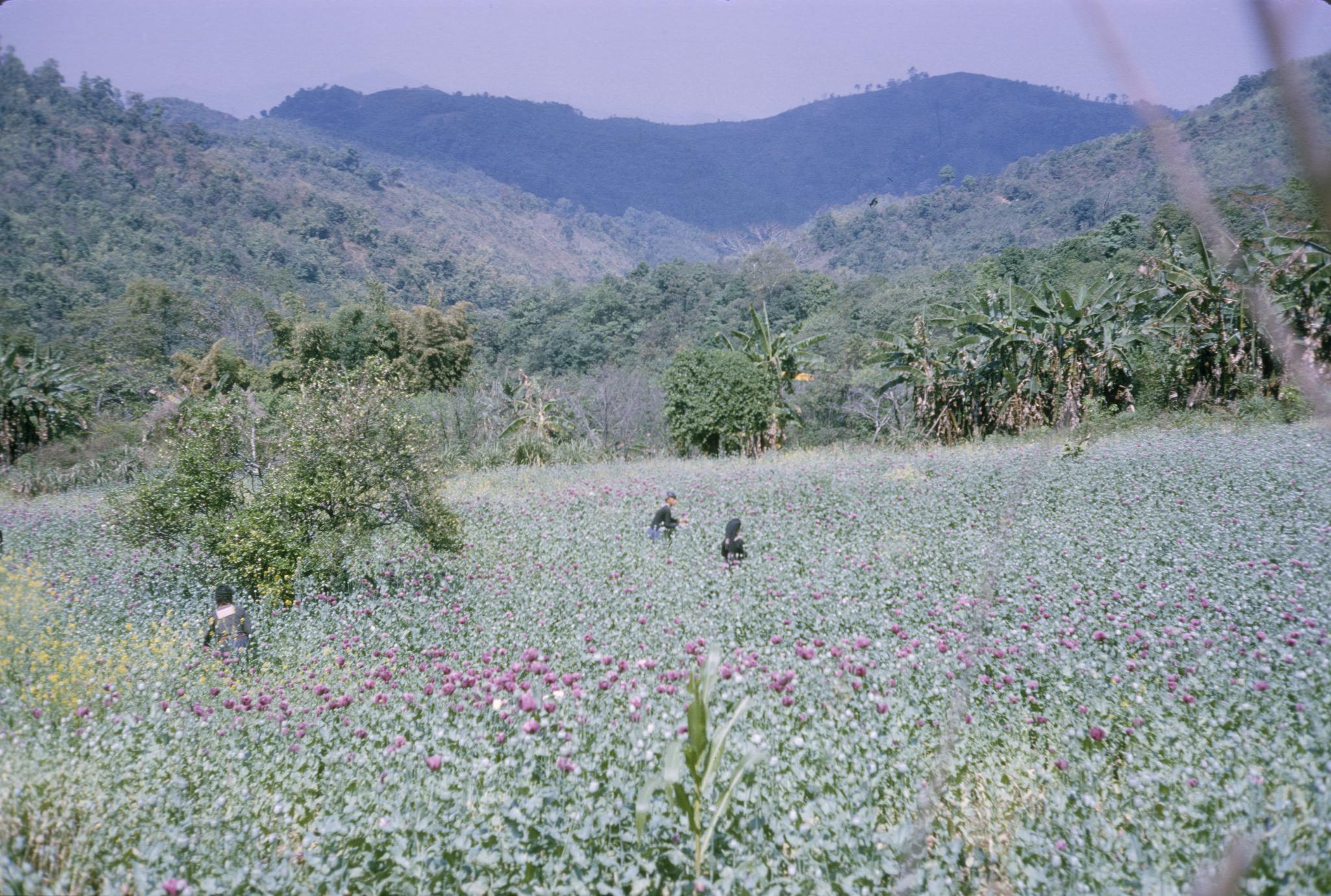The image depicts a vast, rectangular field of tall, green plants reaching nearly shoulder height, dotted with an abundance of purple and some red flowers. Three people are discernible in the field, each clad in black attire with head coverings. Two of them stand close together in the center, while the third person is slightly distanced to the left. In the background, a collection of green and brown-leafed trees stretches out towards large, rolling hills covered in lush, green vegetation. The hills transition into a distant mountainous terrain shrouded in a hazy, dark green hue. Above, the sky presents a unique shade of purple. At the top right corner, part of a plant stalk is visible, adding to the intricate natural details captured in this outdoor photograph.